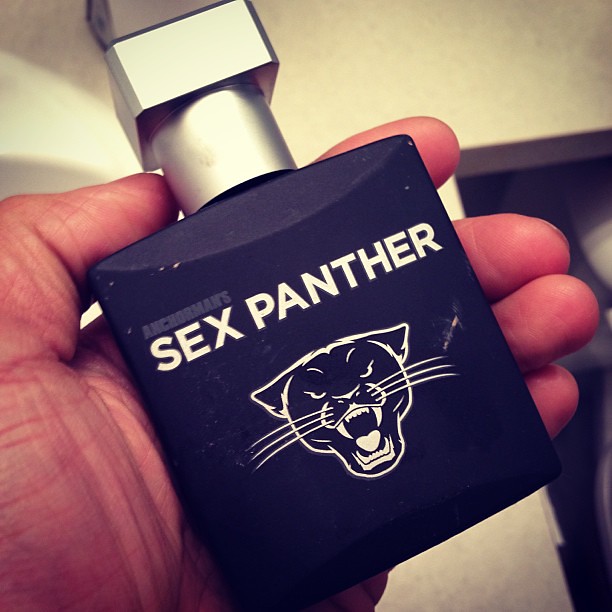This color photograph showcases a dark, angled bottle of grooming product labeled "Sex Panther" in white text on the front, with the word "Anchorman's" in light purple above it. The bottle features an outline illustration of a snarling cougar’s face with its fangs and whiskers prominently displayed. The bottle, which has a silver cap, is being held upright in the palm of a person's hand, with the hand appearing to be that of a man's. The background is a lightly cream-colored, indistinct room, with an empty, dark doorway visible. The photograph is in a square format and illustrates a sense of realism and product photography.